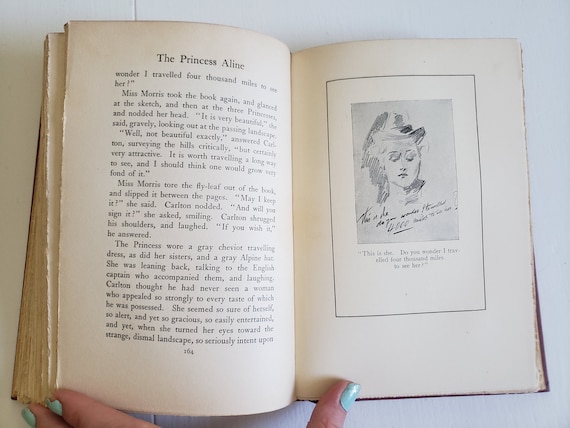The image shows an open, weathered book held open by a left hand with short, light blue polished nails, positioned in the lower left corner. The book is open to page 264, with aged, yellowish-tan pages. On the right page, titled "The Princess Aline," there are four full paragraphs written in black font, with the top of the page featuring a sentence fragment. Below that is a rectangular sketch of a woman with uplifted hair, enclosed in a smaller gray rectangle. There are inscriptions both within and beneath the sketch. The left page contains continuous text, and the entire scene is set against a white background, highlighting the book's aged and worn condition.